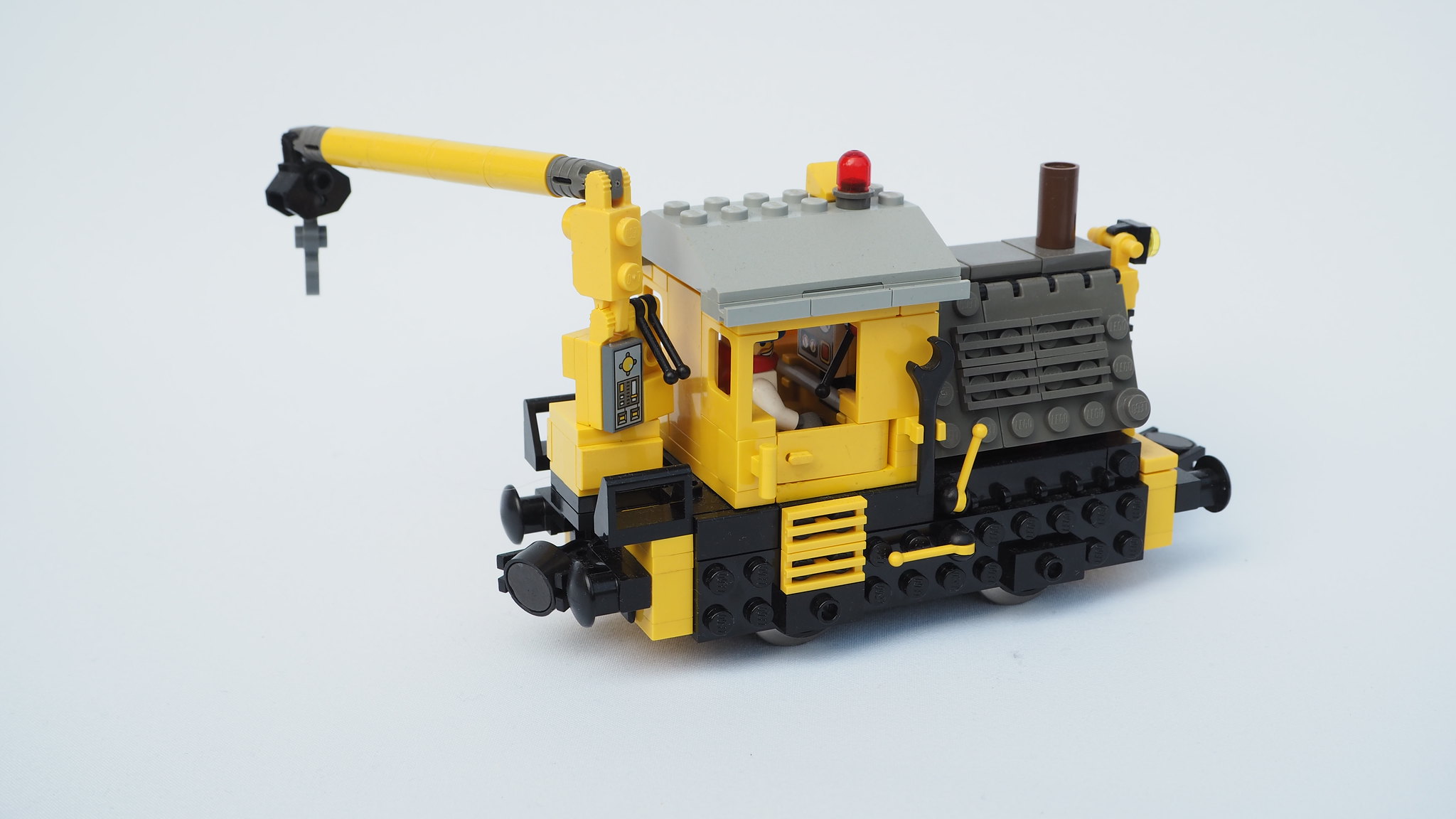The image showcases a detailed Lego construction vehicle that appears to be a hybrid between a crane and a train engine. The vehicle features a swing arm with a hook extending from the rear and a small smokestack at the front, suggesting elements of both construction and rail machinery. Predominantly yellow and gray with black accents, the vehicle includes a small worker figure visible inside. The photograph, likely taken on a white table against a gray or white backdrop, captures the vehicle at an angle that reveals its side and front, offering a clear view of its intricate Lego construction. The overall setting enhances the vivid contrast and detail of the Lego model, which seems professionally staged, possibly for a product display or sale.